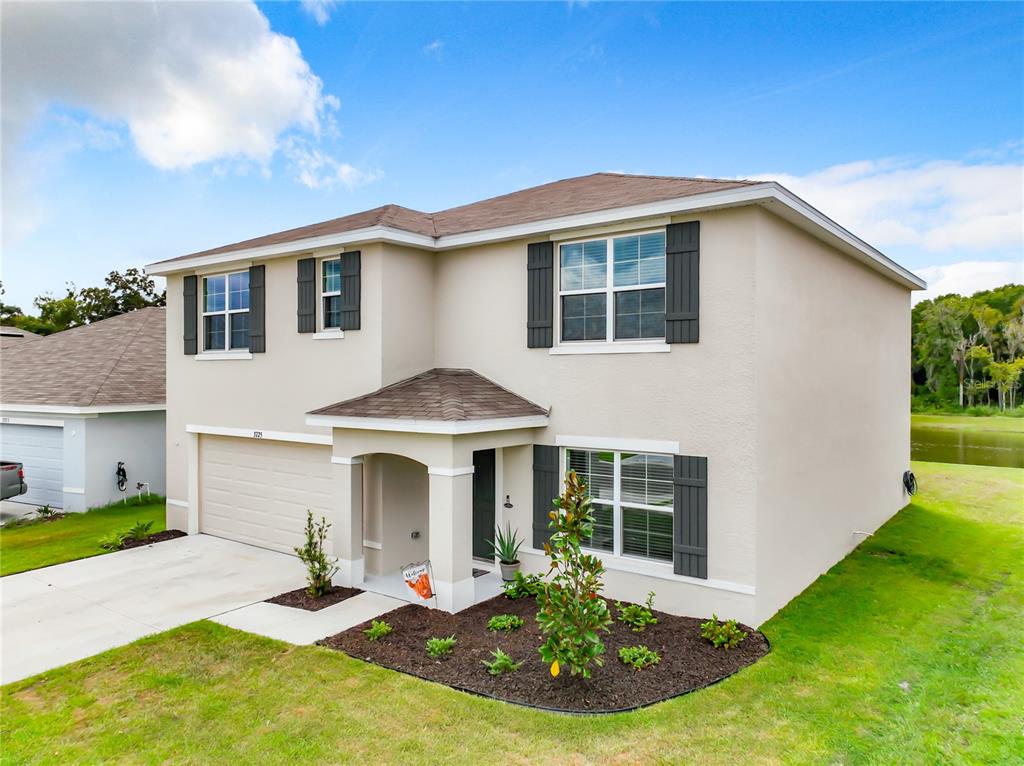The photograph showcases a charming two-story suburban house with a beige or light pink exterior and a copper-colored roof. The front entrance is adorned with a small covered porch supported by a couple of pillars and featuring a copper roof, matching the house's main roof. The house includes a total of four visible windows; three upstairs and one downstairs, all with green shutters. The main floor window is large and flanked by shutters, directly above it there's another similar window, and a same-sized window above the garage. Additionally, a smaller window, presumed to be for the bathroom, is also present upstairs.

The front door, painted green, opens to a small foyer, leading to a well-maintained garden filled with soil. The garden is situated before a concrete driveway, which curves sharply to lead to the garage. Surrounding the house is a neatly trimmed field, and a small body of water, or a little lake, is visible behind the house. The sky above is bright blue with a scattering of fine white clouds. The environment hints at a peaceful vibe where children might enjoy fishing or swimming in the lake. While the home has a cozy and inviting feel, it is relatively close to neighboring houses and could benefit from the addition of a few trees or bushes for added privacy.